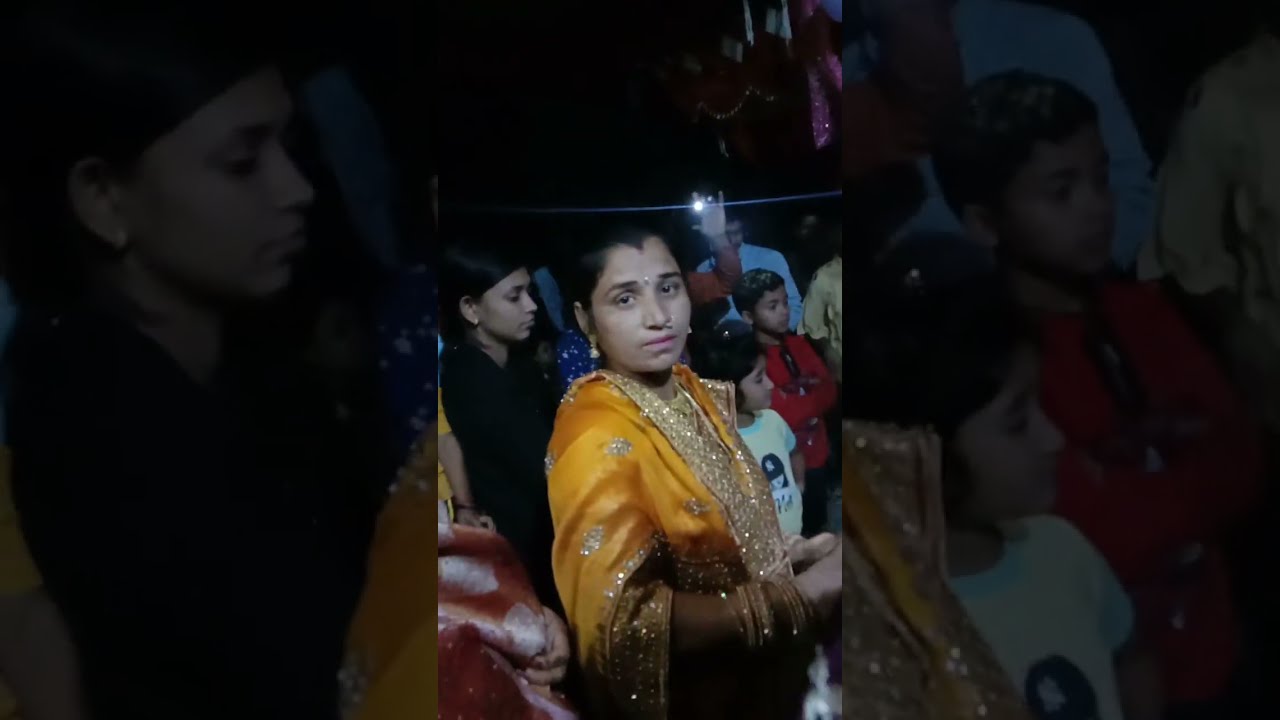The image is a composite divided into three vertical sections, with the outer sections being darkened and enlarged close-ups of the central photograph. The central image, captured outdoors at night, features a group of Indian individuals. The focal point is a woman with black hair, featuring a strong widow’s peak and pulled back, who is staring directly at the camera. She is adorned in a yellow traditional saree with golden, shiny borders on the sleeves, complemented by long, dangly earrings, a pearl on her forehead, and a winged nose piercing. Surrounding her are a few Indian children, including a young girl in a black dress and a little boy, both looking away from the camera. To the right, behind the woman, a hand is raised, possibly holding a phone with its flashlight on, emitting a shiny ray of light. The event occurs under a completely dark sky, reinforcing the nighttime setting.